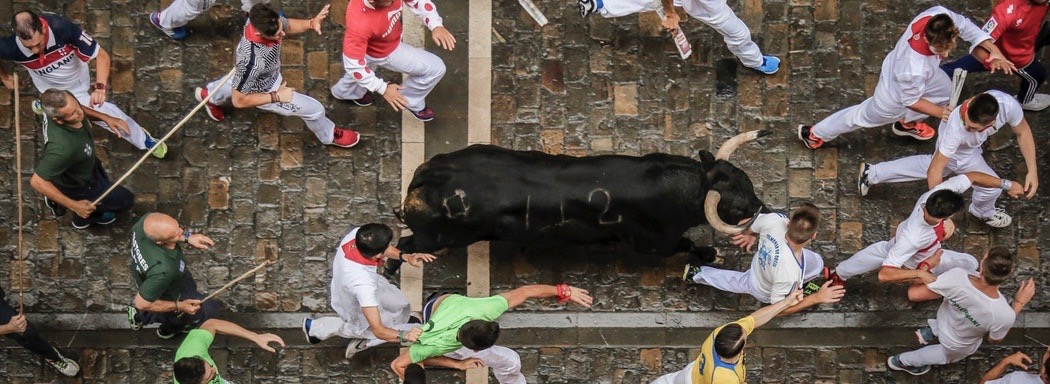The photograph captures a dynamic scene from an aerial, drone perspective, showcasing a black bull with large, curved beige horns running through a street. The bull, which has an illegible number branded or stenciled on its side, is pictured moving towards the right side of the image. Surrounding the bull are numerous people, many of whom are dressed in white shirts and pants, suggestively in a state of pursuit or evasion. Among them, two men in gray jumpsuits are seen carrying long brown sticks or prods, likely attempting to control or guide the bull. The street underfoot displays a pattern of grey and brown tiles or cobblestones, adding texture to the scene. The image, characterized by photographic realism, effectively conveys the motion and urgency of the moment, with one person notably close to the bull's horn near the lower right corner of the frame.